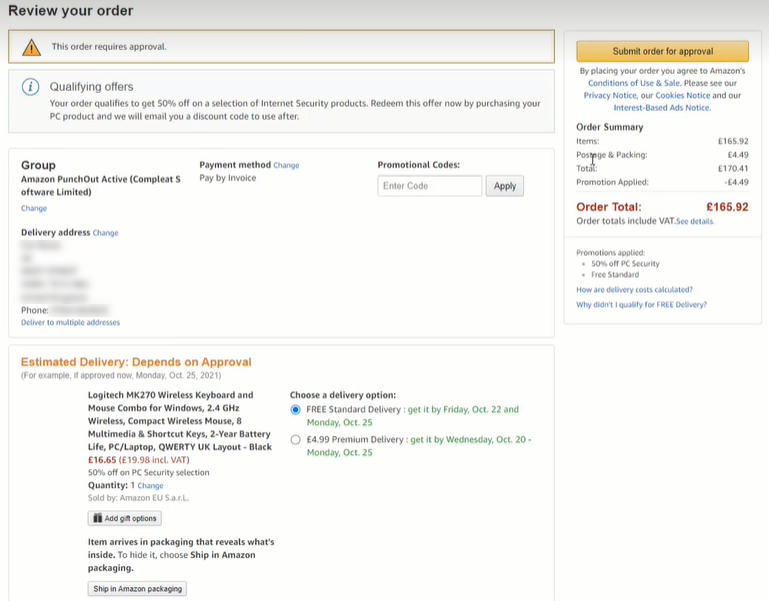This image captures a screenshot of an Amazon.com order review page. The interface features a clean, white background with the headline "Review Your Order" prominently displayed at the top left. Beneath the headline, a cautionary note states: "Caution: This order requires approval." It is followed by a promotional message explaining that the order qualifies for a 50% discount on selected internet security products. To redeem this offer, the customer must purchase a PC product, after which a discount code will be emailed.

Further down, there are sections detailing various order attributes. The "Group Amazon Punch Out" status reads "Active/Complete," and the "Software Limited" designation is noted. The payment method listed is "Pay by Invoice." There is a section for promotional codes, which precedes the "Delivery Address" field—this field, along with the associated phone number, is blurred for privacy. Options to "Deliver to multiple addresses" or to "Change your delivery address" are provided as clickable links.

The estimated delivery date is indicated as contingent upon approval, with an example date given as Monday, October 25, 2021, if approved immediately. The product in question is listed as the "Logitech MK270 Wireless Keyboard and Mouse Combo for Windows," priced at $16.65 with an added note about the 50% discount on PC security products. The shipping method chosen is "Free Standard Delivery."

On the right side of the screenshot, there's a prominent button titled "Submit Order for Approval." The order summary below it shows a total cost of $165.92, and a link to submit the order for approval is provided.

Overall, the image reflects a detailed and clearly organized Amazon order review interface, capturing all necessary elements for the customer to make any final adjustments before submitting their order for approval.